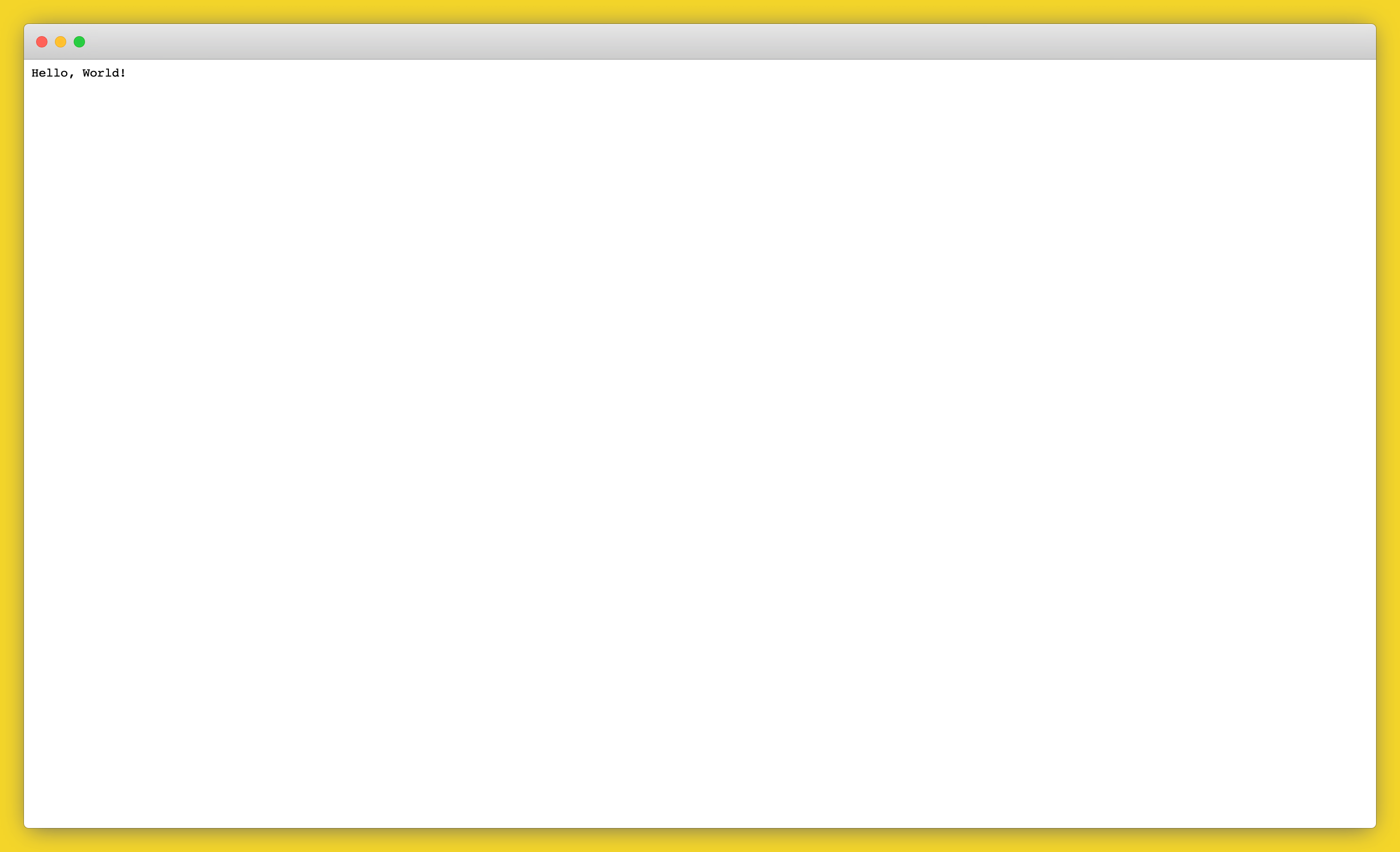Detailed Caption:

The image features a predominantly blank screen with a minimalist design. At the very top of the screen, a subtle light gray background spans from edge to edge, providing a calm backdrop. In the top left corner, there are three small dots arranged horizontally: a red dot on the left, followed by a yellow dot in the center, and a green dot on the right. Below these dots, in the same top left corner but slightly lower, there's a tiny black text that reads "hello, world..." The entire screen is bordered by a thin yellow square, framing the minimalist content and adding a touch of vibrant color to the otherwise simple composition. This yellow border completes the overall image.